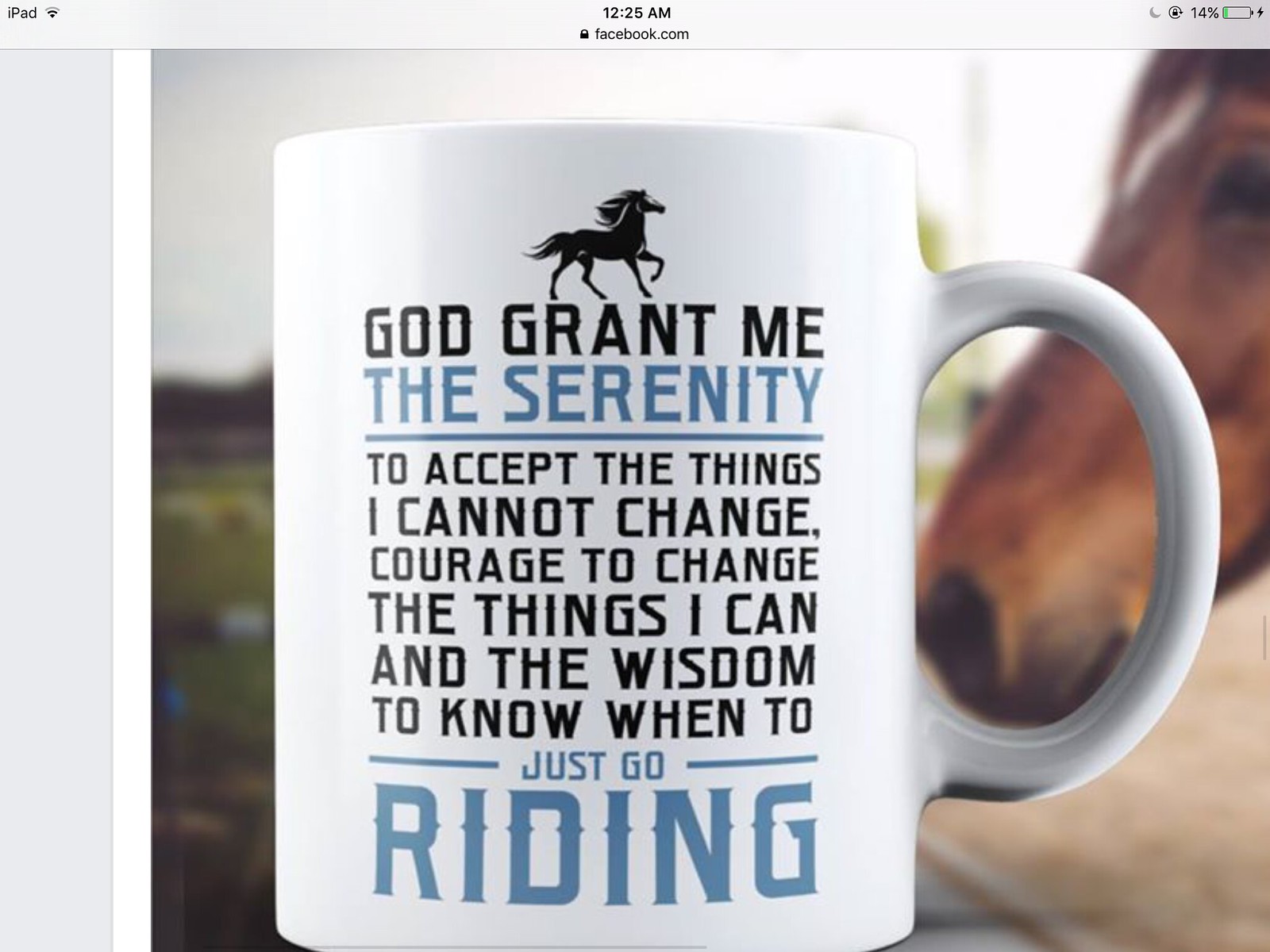The image is a detailed screenshot from an iPad, captured at 12:25 a.m., with a battery level of 14%, showing a Facebook post of a distinctive white mug. The mug features a combination of black and blue text with an elegant layout. At the top, in black text, it says, "God grant me," followed by a black clipart image of a horse. Below, in blue text, it reads "the serenity," underlined for emphasis. A paragraph in black text continues with the words, "to accept the things I cannot change, courage to change the things I can, and the wisdom to know when to," followed by "just go riding" in blue text. To the right edge of the image, partially in the background, a horse's head is visible, bearing a brown coat with a distinctive white patch on its forehead. The image, taken outdoors in clear lighting, encapsulates a tranquil message and setting.